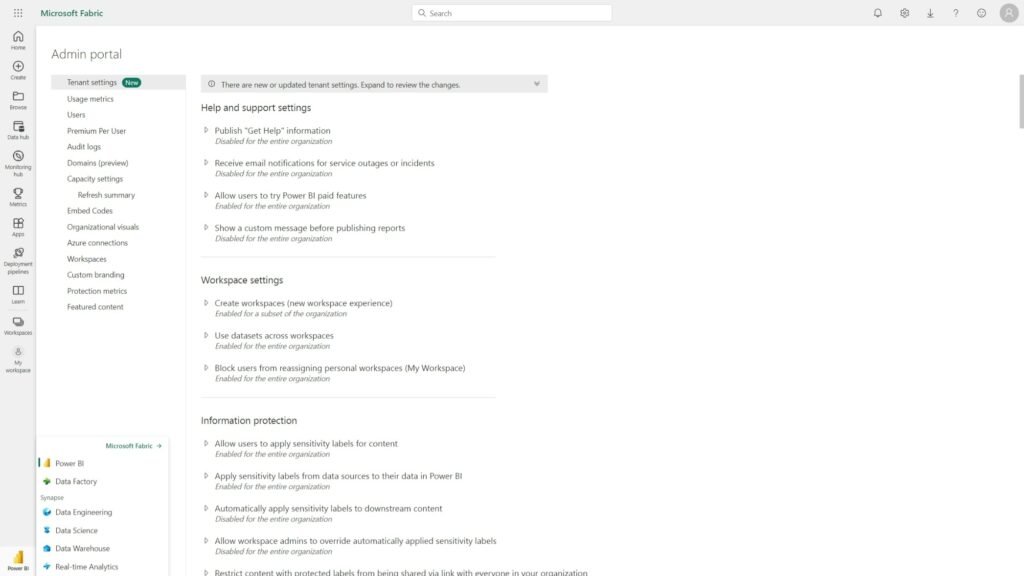The image showcases a user interface for "Microsoft Fabric." At the top of the screen, the title "Microsoft Fabric" is prominently displayed alongside a search bar. On the left side of the screen, there is a sidebar featuring various icons, with the home icon being the most identifiable one.

Despite some blurriness obscuring parts of the image, specific sections of the interface are clear. To the right, headers such as "Admin Portal" and "Tenant Settings" stand out. Beneath these, a list of categories is visible, including Usage Metrics, Users, Premium Per User, Audit Logs, and Domains. Other manageable sections include Preview, Capacity Settings, Refresh Summary, Embed Codes, Organizational Settings, Workspaces, Custom Branding, Protection Metrics, and Featured Content.

Additionally, on the right side of the interface, there is a "Help and Support" section followed by Settings. Though some options under this menu are unclear, other sections such as Workspace Settings and Information Protection are distinctly readable.